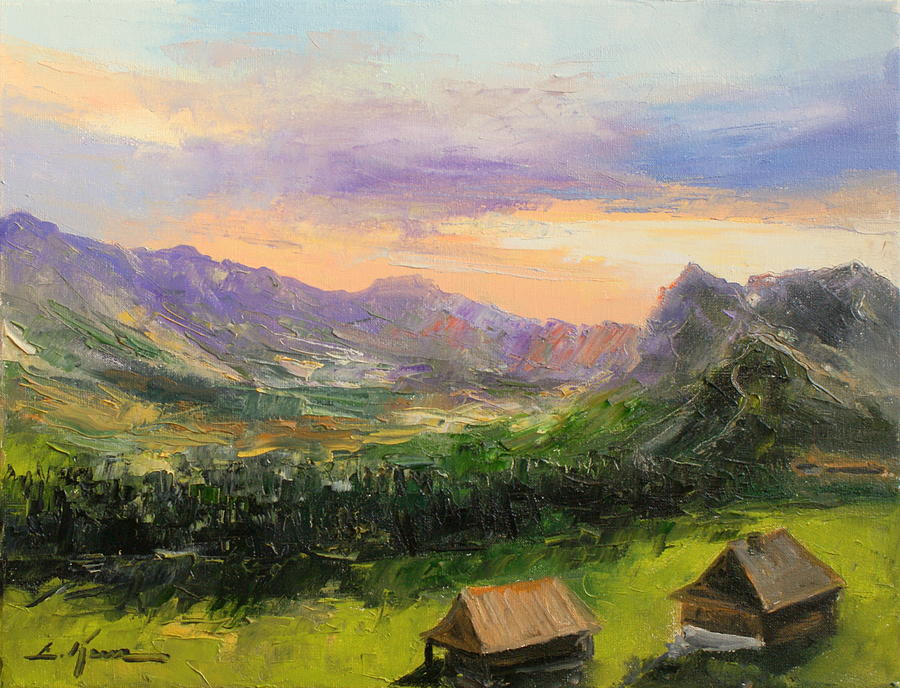This vibrant oil painting captures a serene nature scene at sunset, where the sky transitions from rich lavender at the top to refreshing light yellow closer to the horizon. Dominating the landscape are blue and purple mountains tinged with red, creating a dramatic backdrop. In the midground, a band of dark green trees and foliage contrasts against the mountains, adding depth to the composition.

In the foreground, nestled in lush green grass, are two small wooden cabins resembling log houses. These cabins, one in light-colored wood and the other in darker wood with white trim, both feature raised foundations and inviting porches. Between the mountains and the cabins, a clear blue brook or stream meanders through the scene, reflecting the sky.

The bottom left corner of the painting is marked by the artist's signature, possibly starting with an "L" followed by a "K" and some illegible squiggles, adding a personal touch to this picturesque artwork.